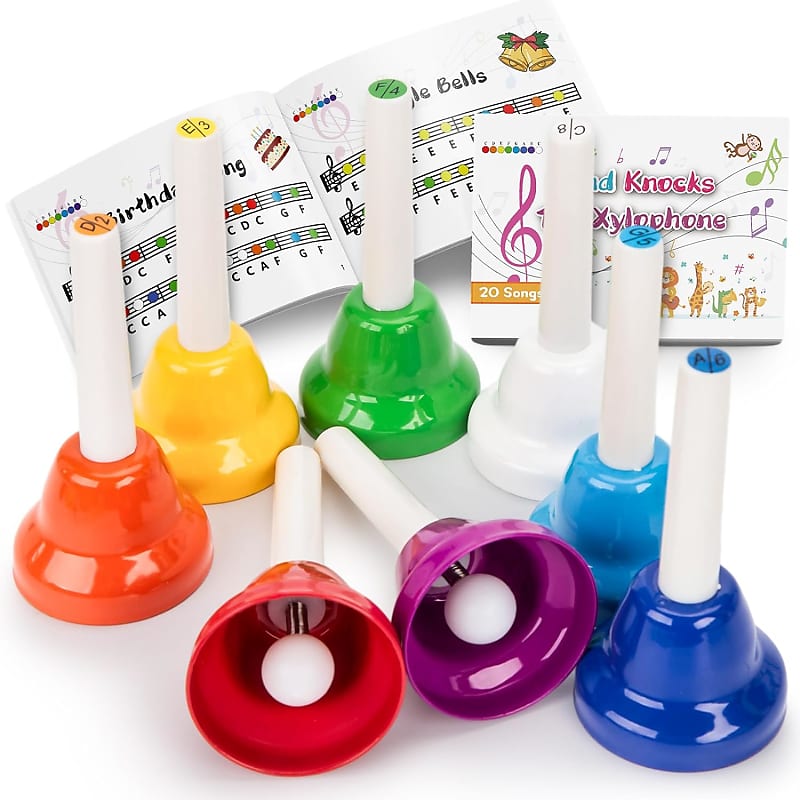This image showcases a colorful set of eight small handbells, each with a white stem and uniquely colored base: orange, yellow, green, white, light blue, royal blue, red, and purple. Arranged neatly on a table, these bells are labeled with musical notes such as D2, E3, F4, C8, G5, and A6. In the backdrop, against a clean white background, lie two instructional booklets. One booklet appears to guide the user through 20 songs, including "Happy Birthday" and "Jingle Bells," with indications on which bell colors to use for each note, represented visually with musical notes and corresponding colored sections. The second booklet, partially visible, mentions a xylophone and further song instructions. This indoor setting highlights the educational and playful nature of the musical toy set designed for children.